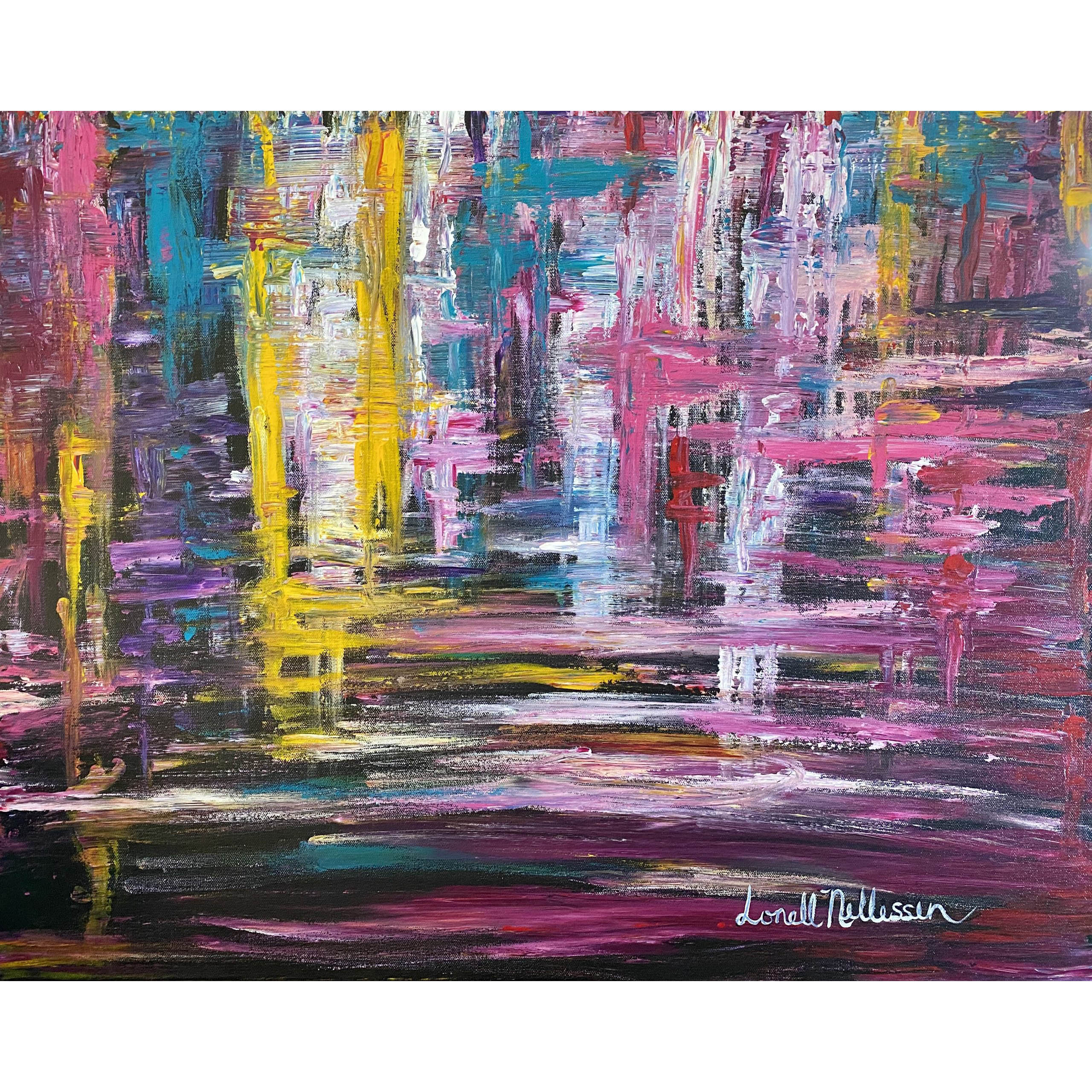This image is a vibrant and captivating piece of modern art known as "Times Square Puddle" by artist Lonell Nellison. The original painting measures 24 inches by 30 inches, making it a substantial piece of artwork. Executed in a highly abstract style, the painting showcases a dazzling array of colors and textures reminiscent of the myriad lights reflecting off a wet street at Times Square.

In the bottom half of the artwork, the colors are arranged in horizontal stripes featuring reds, blues, blacks, and dark shadowy hues, with occasional highlights of white. This section is notably darker and appears to have been created with thick, textured strokes, possibly using a palette knife. As the painting progresses upwards, the stripes transition to a vertical orientation, blending into a lighter palette with more whites, yellows, reds, and blues. 

The left side of the image is especially dynamic, with a diagonal composition moving from darker tones at the bottom to lighter and more varied colors at the top. There are patches of purple, blue, green, and yellow, each adding depth and contrast to the overall composition. On the right side, the colors take on a warmer tone with reds, pinks, and purples creating a lively interplay with the rest of the artwork.

A distinguishing feature of the painting is the artist's signature in the bottom right-hand corner, written in white cursive and reading "Lonell Nellison." This detail provides authenticity and a personal touch to the piece. The combination of varied textures, colors, and the abstract representation of lights makes this artwork an enchanting and thought-provoking visual experience.